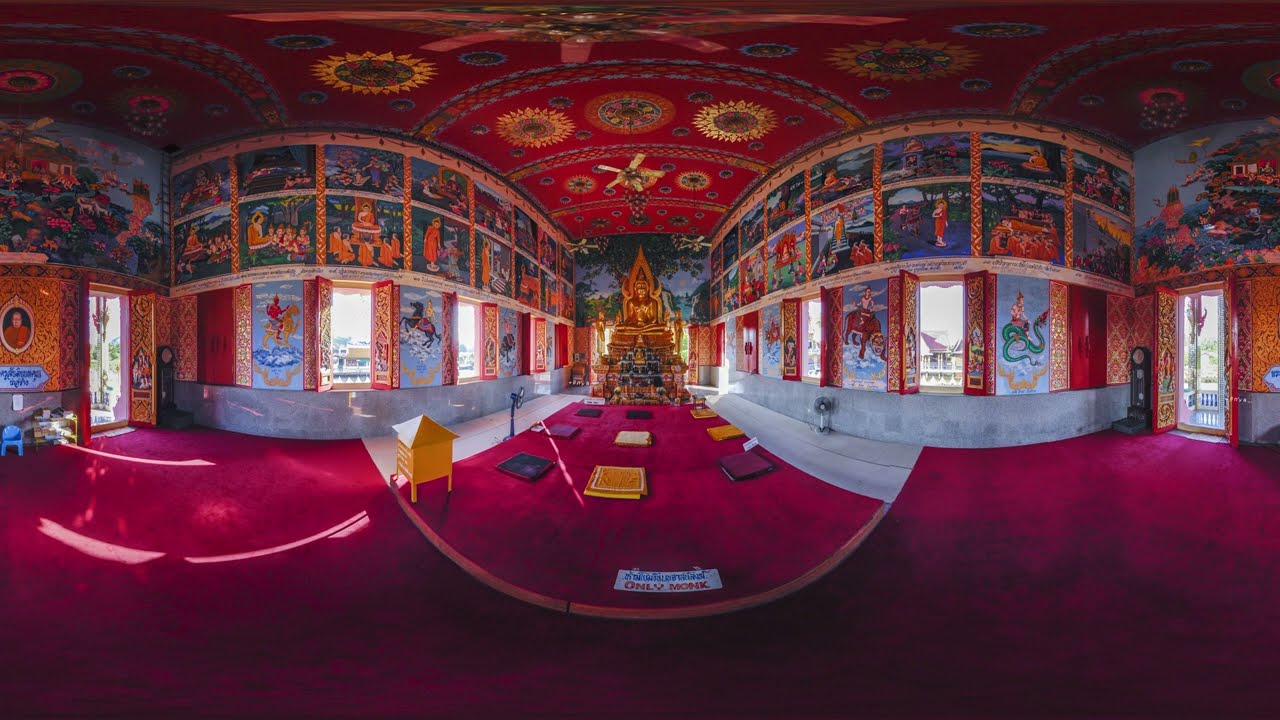The photograph captures the opulent and intricately designed interior of a temple, possibly Hindu or Buddhist, distinguished by a vibrant color palette of purple, red, and gold. At the center of the temple, a resplendent golden statue stands majestically, possibly depicting a deity or Buddha, surrounded by books neatly arranged on a vivid purple carpet. The walls of the room soar high, adorned with elaborate, story-telling murals featuring scenes like a snake, an elephant, a rhinoceros, and a horseback rider. The room's highly detailed ceiling, painted in a burgundy and gold pattern that mimics Persian rug designs, adds to the ornate ambiance. The structure includes arched doorways and windows with red and gold shutters that allow glimpses of a clear, bright blue sky outside. Across the fuchsia pink carpet on the floor lie an assortment of prayer mats and square-shaped pillows in gold, fuchsia, and blue, enhancing the room's colorful appearance. The entire panorama is captured in a 360-degree image, which lends a warped, curvilinear perspective to the scene, intensifying the sense of grandeur and intricate detail.